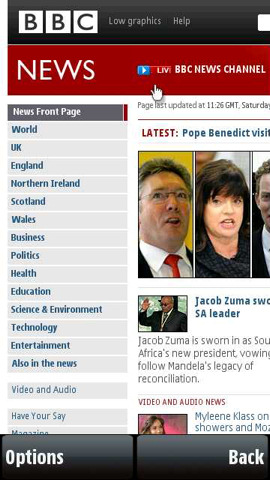This is a screenshot from a mobile device showcasing a BBC news page. In the upper left-hand corner, the iconic BBC logo, represented by the letters "BBC" within squares, is prominently displayed. Adjacent to the logo are the options "Low Graphics" and "Help." The top banner of the page is gray, below which is a red banner labeled "News" in large white text, accompanied by the title "BBC News Channel."

On the left side of the image, a dropdown menu labeled "News Front Page" is highlighted. To the right of this menu, the screen displays an article titled "Latest: Pope Benedict," followed by three vertical portrait photos. Beneath these photos is another article titled "Jacob Zuma as a Leader." The left vertical section offers a navigation menu listing categories such as News Front Page, World, UK, England, Northern Ireland, Scotland, Wales, Business, Politics, Health, Education, Science & Environment, Technology, Entertainment, and Also in the News. Additionally, it includes sections for "Video & Audio" and "Have Your Say."

The bottom of the screen features a large footer with two gradient-colored buttons. The button on the left reads "Options," while the button in the right bottom corner is labeled "Back."